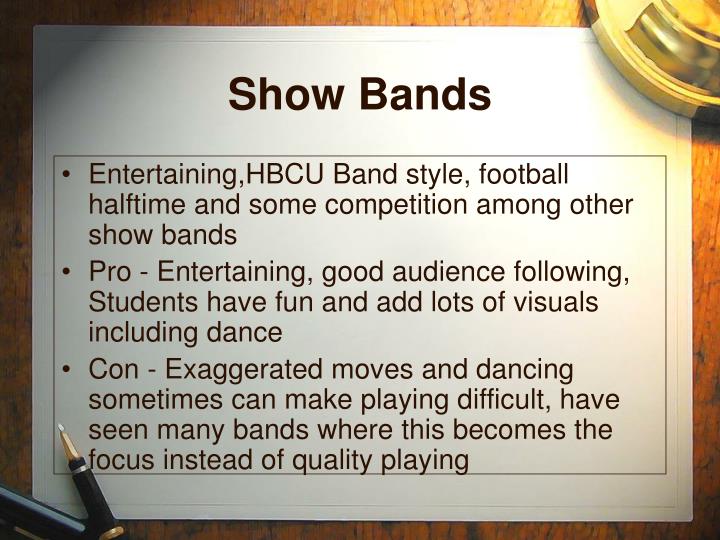This image features a brown table with a white printout of a PowerPoint slide laying on it. The slide is titled "Show Bands" in black text. Within a black-bordered section, three bullet points describe various aspects of show bands. The first bullet point states, "Entertaining HBCU band style, football halftime, and some competition among other show bands." The second bullet point, labeled "Pro," mentions that show bands are "entertaining, have a good audience following, students have fun, and add lots of visuals including dance." The third bullet point, labeled "Con," notes that "exaggerated moves and dancing sometimes can make playing difficult," and it adds that in many bands this becomes the focus instead of quality playing. In the lower left-hand corner of the table, there is a section of a gold lamp base and two pens—one with its cap off, lying at an angle. The paper also appears to be held down by a paperweight on the right side, completing the detailed snapshot of this desk scene.